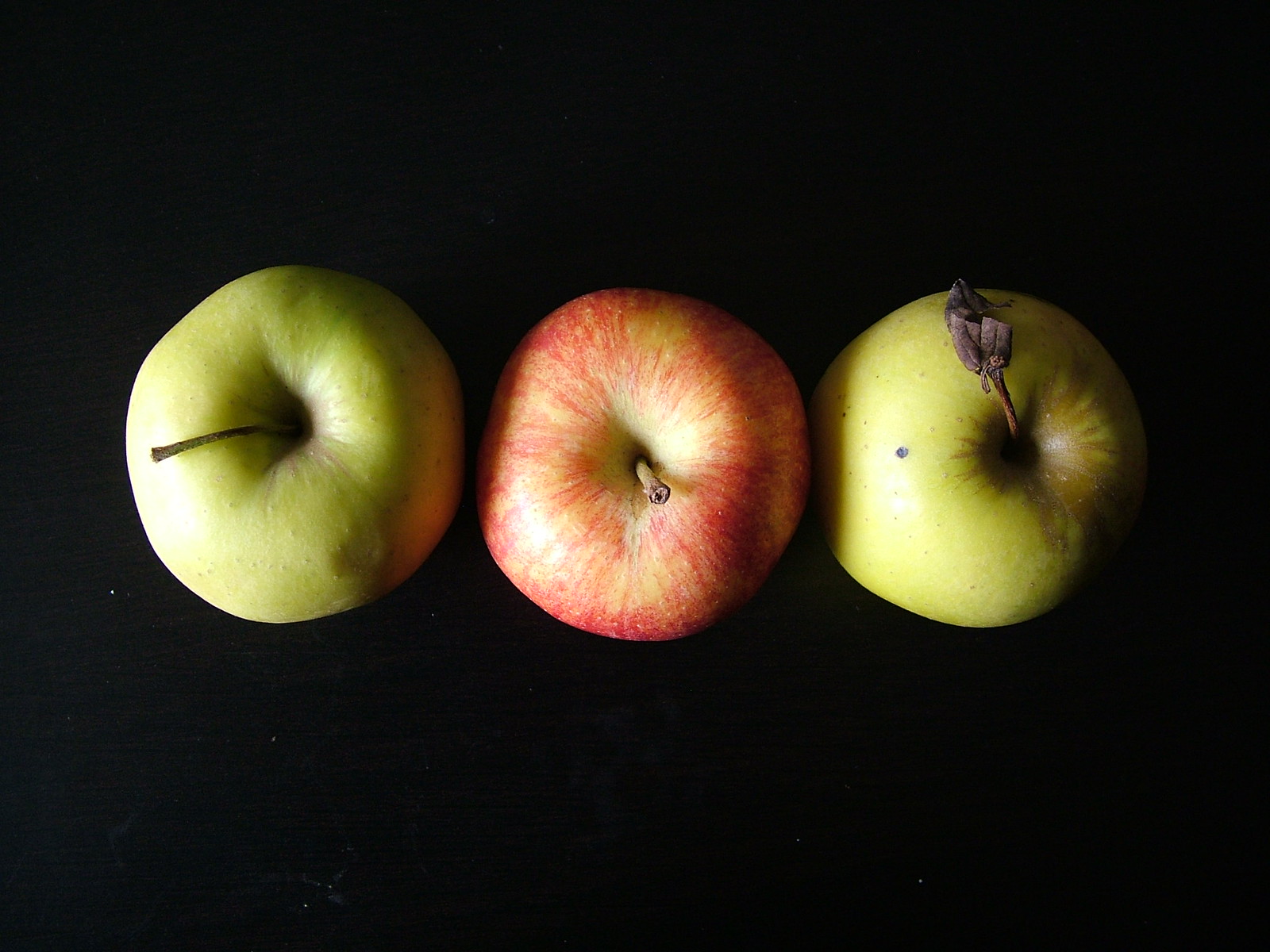This image portrays a top-down view of three apples aligned in a straight row against a completely black background. The two green apples bookend a singular red apple that exhibits yellow streaks. All three apples retain their stems, with the green apple on the right featuring a withered, brown leaf at the tip of its stem. The leaf appears curled and lifeless, set at an angle pointing roughly toward the 11 o'clock position. Each apple casts a shadow toward the right, indicating light striking from the left side of the frame. Additionally, the green apple on the right shows a hint of browning around its center.